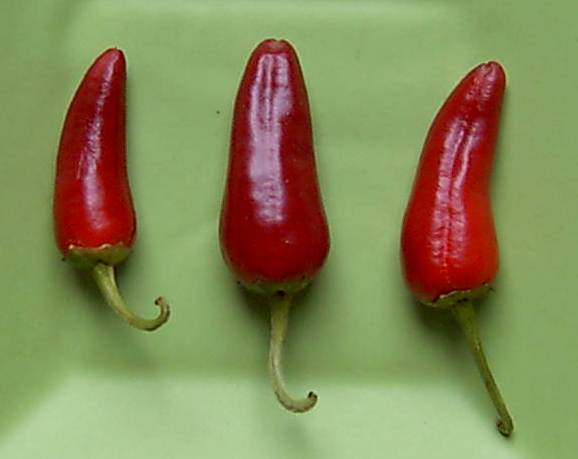This photograph features three red chili peppers arranged side by side on a light green rectangular plate with a subtly sloping center. The left-most pepper, being the smallest, has a slightly wrinkled top and its light green stem curls up to the left. The middle pepper, the largest and roundest of the three, boasts a deep maroon hue with a shiny, speckled surface. Its stem curves upward and slightly to the right. The right-most pepper is lighter in color and has a straight stem that points downward. Each pepper's shape resembles that of a jalapeno, with the ones on the outside having more noticeable curvature. The background, an olive-green dish transitioning to a lighter green towards the bottom, adds a complementary contrast to the vibrant red peppers.